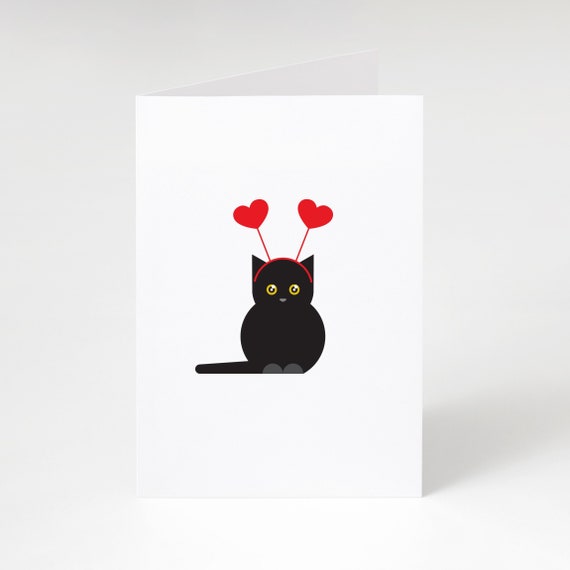The image depicts an illustrated greeting card standing upright with its spine on the left. The entire scene is set against a solid white background, and the card itself is made of white paper. The focal point of the card is a charming, chubby black cat whose body and head are almost perfect circles. The cat features shiny yellow eyes gazing straight ahead, a small gray nose, and pointy triangular ears. Two gray paws are visible in front of its body, while its tail lies flat on the ground to the left. Adding to the cat's whimsical appearance, it wears a red headband with two antennae ending in bright red hearts. The illustration exudes a playful and cutesy vibe, and the overall aesthetic of the card suggests it could be a get-well or a similarly cheerful greeting card.